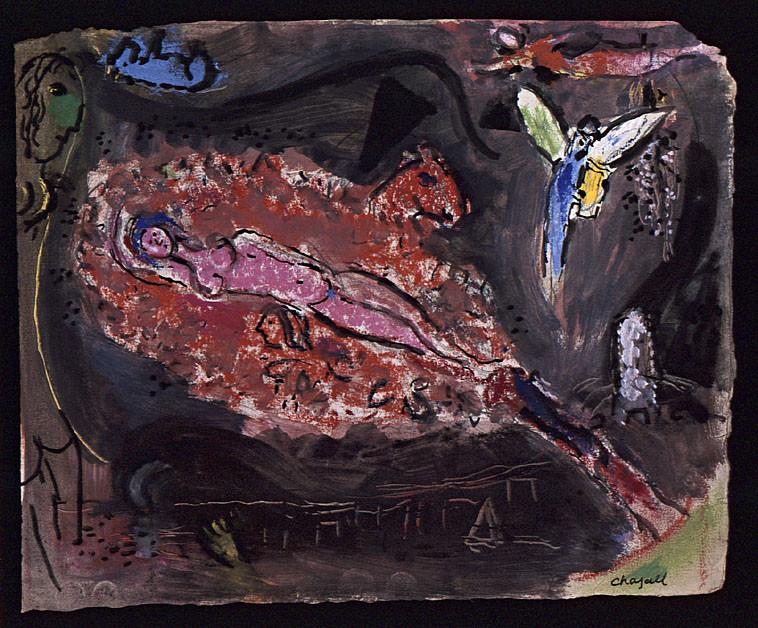The image depicts a large, square painting set against a solid black background, with the painting's edges appearing tattered and uneven, almost as if the paper is ripped. Signed "CHAJALL" in the lower right-hand corner, this vivid and abstract piece centers around a striking red and white area. Dominating this central space is the figure of a naked woman with blue hair, her thin body laying diagonally from the upper left to the bottom right. Beneath her in the red section, a profile of a person's face is faintly visible, as well as what seems to be a horse's face towards the upper right.

The surrounding areas of the painting, filled with dark gray and dark blue hues, further branch into intricate, abstract elements. On the upper right, a woman with brown hair and a white face, dressed in red, appears to be flying horizontally. Below this flying figure, an angel adorned with multicolored wings—green and white, and blue and white—holds a yellow object in her hands. The composition includes curved lines, a triangle, and other shapes adding to its confusion and complexity. Toward the upper left, next to the resting woman’s head, another animal figure in blue is subtly outlined.

Overall, this abstract painting melds an array of colors—including black, gray, red, blue, green, and splashes of yellow—into an enigmatic array of figures, faces, and forms, blending them into a surreal narrative that is open to interpretation.